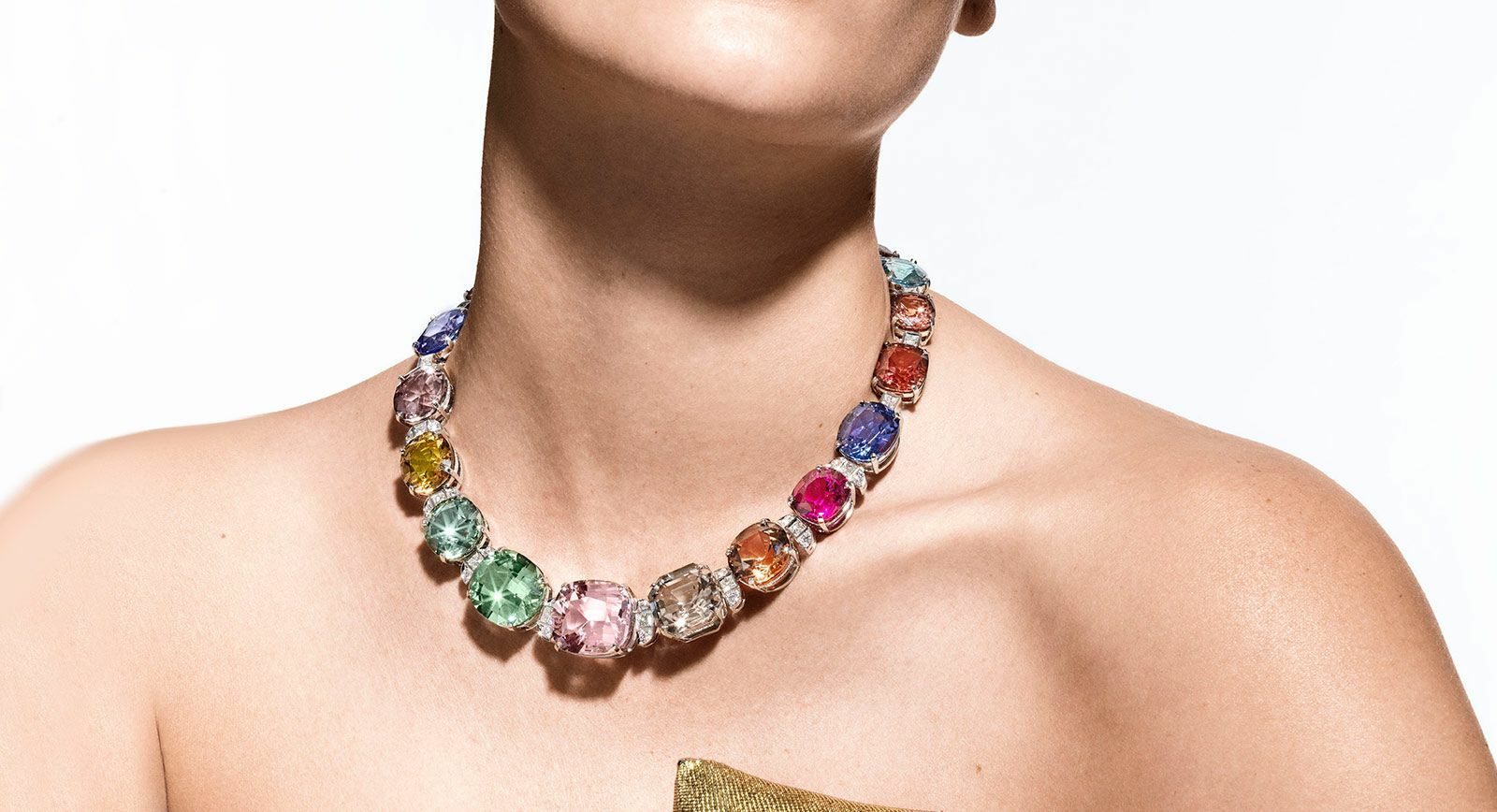This photograph showcases the neck and shoulders of a Caucasian woman whose face is mostly cropped out, displaying only her chin and a hint of her left ear. She is adorned with a strikingly colorful and large necklace, which features an array of gemstones in various shapes — predominantly oval and circular. The necklace includes vivid hues such as emerald green, bright pink, purple, clear, amber, and blue, with each stone being notably larger than an average adult thumb, suggesting they could be precious stones. The necklace consists of approximately 15 to 20 of these substantial stones, arranged closely around her neck. The woman’s bare shoulders and the slight glimpse of a strapless green garment add to the emphasis on the statement jewelry, set against a clean white background.